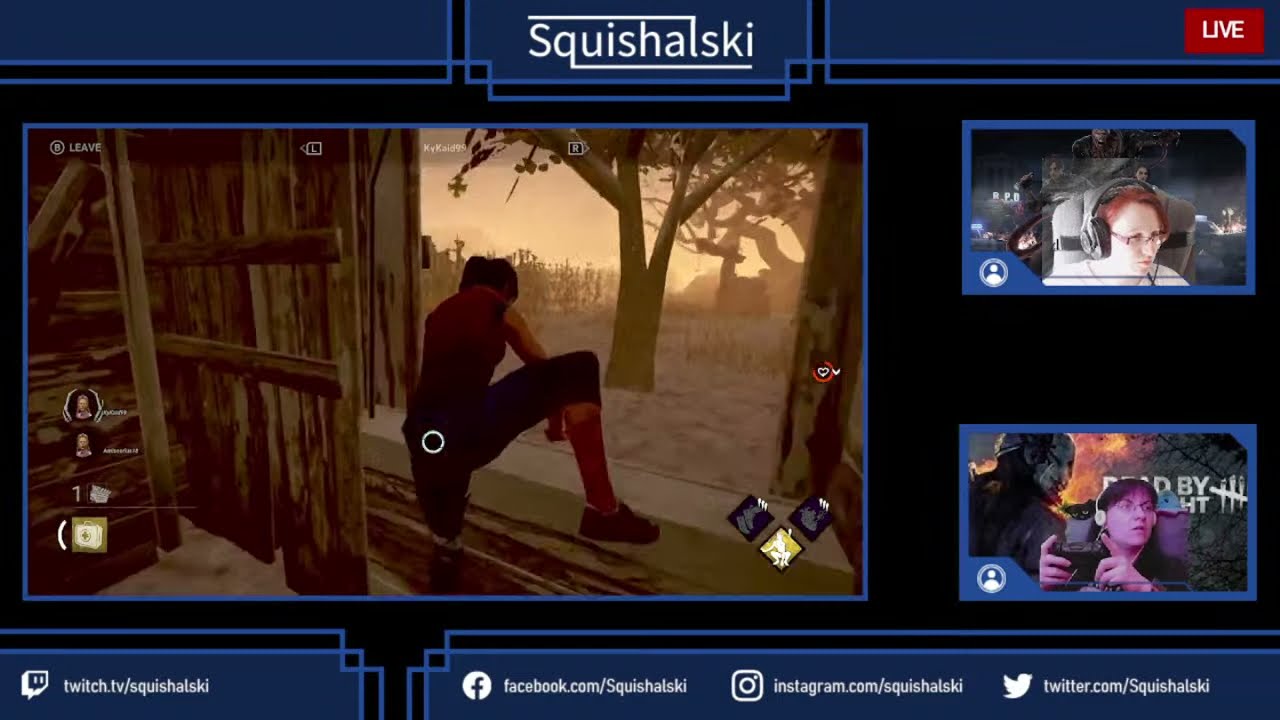This is a detailed screenshot from a live Twitch stream of a multiplayer online video game. The screen is bordered with blue and light blue trim and features multiple visual elements. At the top center, the text "Squishalsky" is displayed in white letters, identifying the streamer. Below, an overlay lists the Twitch URL and social media links for Facebook, Instagram, and Twitter.

The central portion of the screen showcases an in-game scene where a character, dressed in a red shirt, dark pants, and black shoes, appears to be climbing out of a barn window into a foggy landscape with trees, possibly some snow, and a dreary, yellow-tinted sky.

On the right side, there are two webcam feeds of the players. The top feed features a woman with red hair, glasses, and a white shirt, who is wearing a headset. The bottom feed shows another player, ambiguously gendered, with short hair and glasses, holding a game controller. A small red box marked "live" at the top of the screen indicates that this event is being streamed in real-time.

The visual setup and streaming elements suggest an interactive and immersive online gaming experience, likely shared with an audience via Twitch. The game depicted might be a survival title, with some guesses pointing towards "Dead by Daylight" based on the visual context.